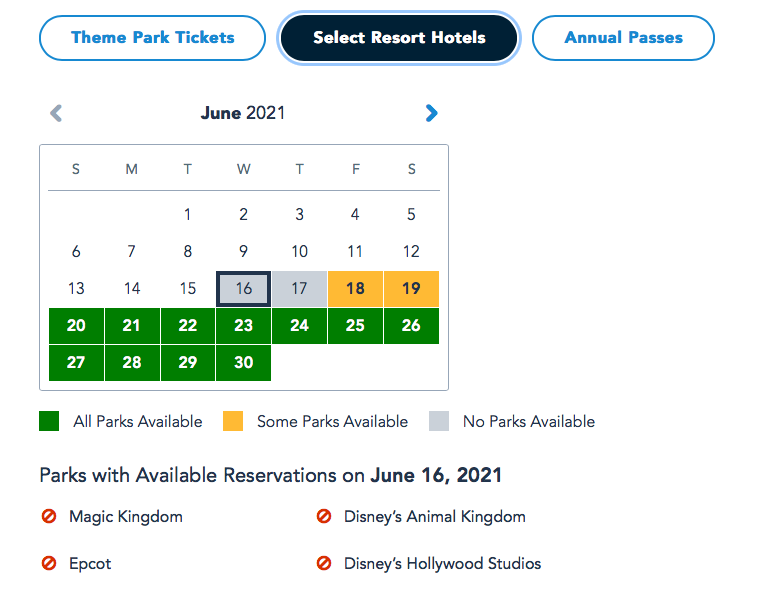Screenshot of a website's selection area showcasing various categories and calendar availability. At the top of the webpage, there are distinct categories listed: "Theme Park Tickets," "Select Resort Hotels," and "Annual Passes." Below these categories, on the left side of the screen, a calendar for June 2021 is displayed. The calendar highlights different availabilities for specific dates: June 20th through June 30th are marked in green, indicating full availability, while June 18th and 19th are highlighted in yellow, suggesting limited availability for these dates.